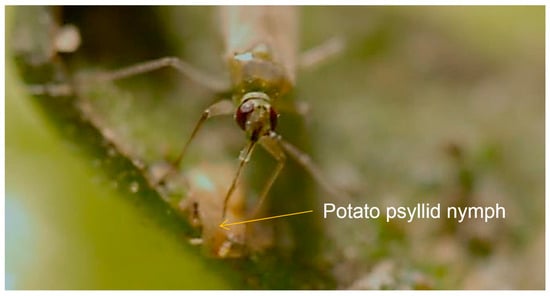This detailed image captures a close-up of a brown, translucent potato psyllid nymph standing on a green leaf. The photo, predominantly green, focuses sharply on the insect's small head, allowing a clear view of its prominent, side-front positioned, burgundy-red eyes. A thin, needle-like proboscis extends from its head, suggestive of its feeding mechanism. The bug, identifiable by its six needle-like legs, has a blurred background that contrasts with its sharp foreground details. A yellow arrow points towards the proboscis, accompanied by white text at the bottom right corner labeling it as "potato psyllid nymph." The bug's unsettling gaze and intricate physical features make it the focal point of the image.